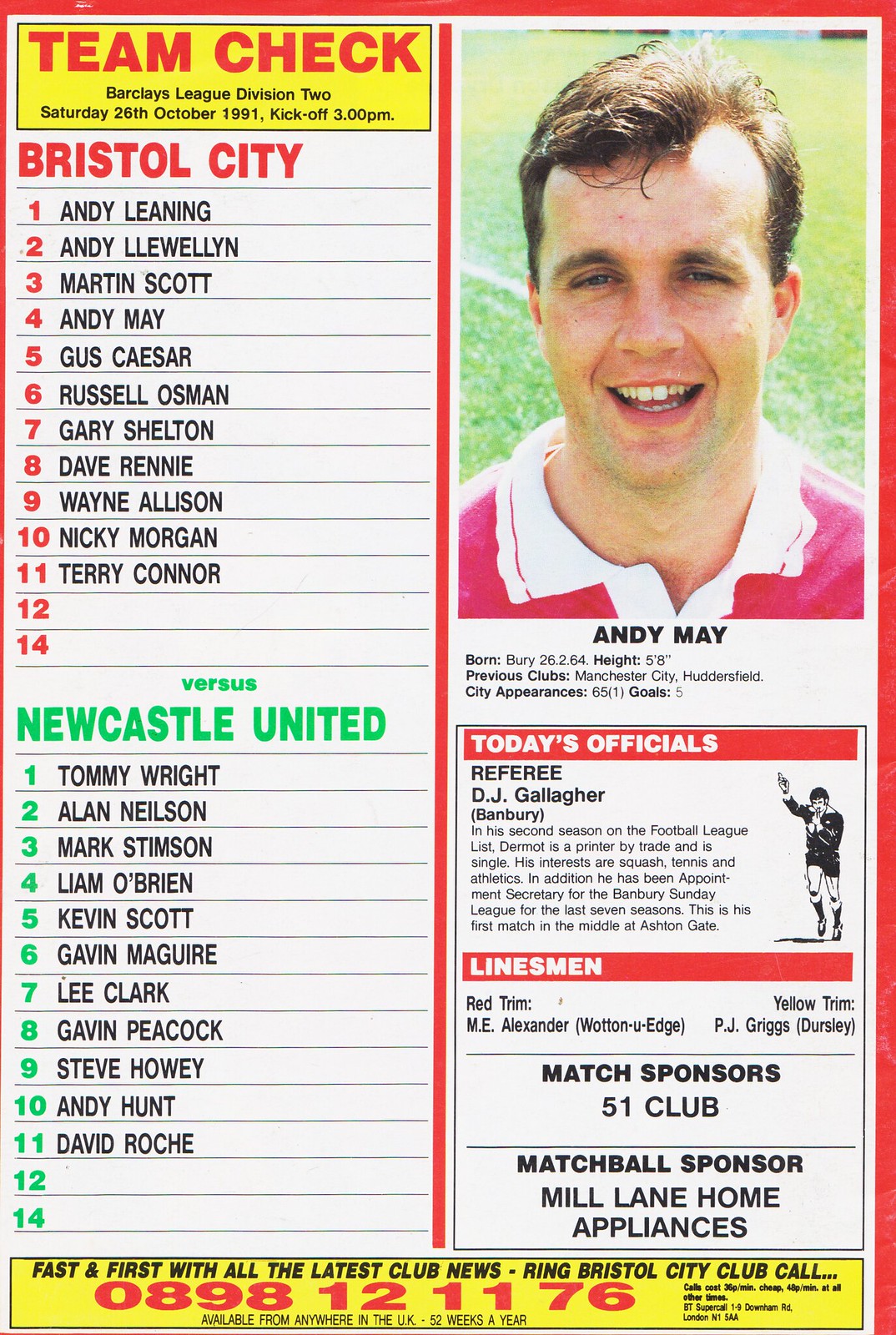The image is a vertically aligned rectangular page from a soccer program, dated Saturday, 26th October 1991, for a Barclays League Division 2 match with a 3 p.m. kickoff. The left-hand side features columns listing the rosters for Bristol City and Newcastle United, with Bristol City players' numbers in red and Newcastle United numbers in lime green. Positioned prominently on the right-hand side is a vertical rectangular photo of Andy May, a soccer player smiling at the camera. He has blue eyes, brown eyebrows, short combed-over brown hair, and is wearing a red jersey with a white collar, against the backdrop of a grassy field.

Details about Andy May are included below his picture: he was born on 26th February 1964 in Barry, is 5'8" tall, and previously played for Manchester City and Huddersfield City, with 65 appearances and 5 goals. The page also highlights the two teams' rosters, including names such as Andy Leaning, Andy Llewellyn, and Martin Scott for Bristol City, and Tommy Wright, Alan Nielsen, and Liam O'Brien for Newcastle United.

Additionally, the program lists today's officials—Referee DJ Gallagher—and the linemen. Sponsor information is provided, naming 51 Club as a match sponsor and Mitch Lane Home Appliances as the match ball sponsor. At the bottom, a yellow banner with red and black text encourages readers to call Bristol City Club at 0898-112-1176 for the latest club news. The overall page design is white with red and green accents, creating a vibrant, detailed visual for fans.